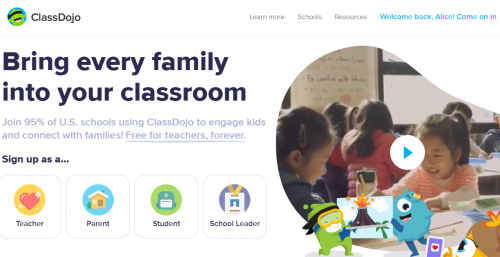This image captures a cropped screenshot of the Class Dojo teacher resource website, set against a clean, white background. Positioned at the top left is the Class Dojo logo. On the top right, a navigation menu displays categories in grey font: "Learn More," "Schools," and "Resources." Further to the right, a personalized greeting reads "Welcome Back, Alice, Come On In" in blue font, indicating that Alice is logged in.

Center stage at the top of the page, bold black letters prominently display the phrase "Bring Every Family Into Your Classroom." Below this in smaller grey text is a call to action: "Join 95% of US schools using Class Dojo to engage kids and connect with families. Free For Teachers Forever," with the latter phrase underlined to highlight its significance.

Beneath this message, a prompt in black font reads "Sign Up As A." Below this prompt, five square icons represent different user types: "Teacher," "Parent," "Student," and "School Leader."

The right side of the page features a small background image of children in a classroom setting, overlaid with a white circle containing a blue play button, inviting viewers to watch a video. Superimposed over the photograph are whimsical cartoon characters, adding an engaging and playful element to the page.